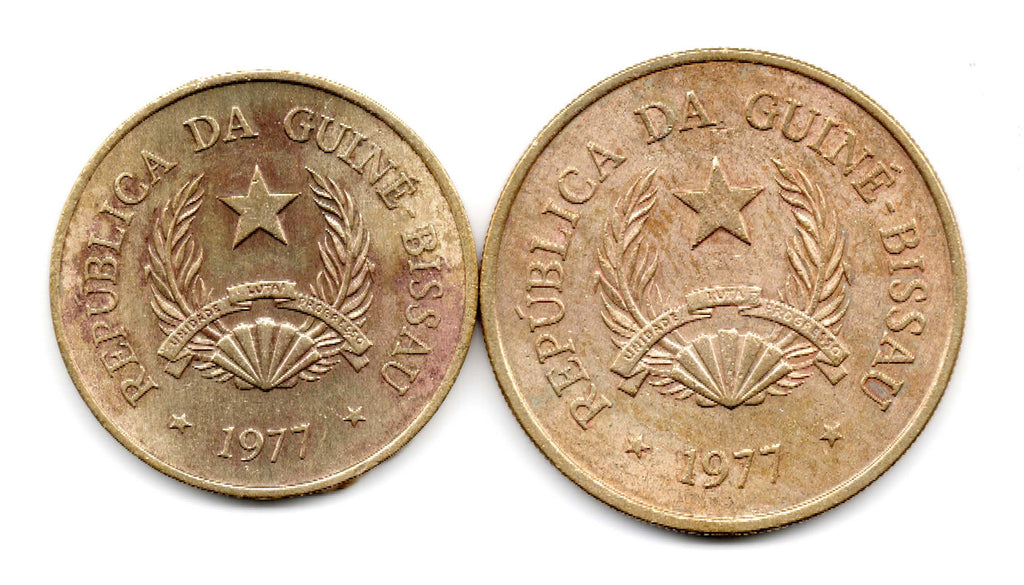The photograph captures two coins, showing both the front and back of the same denomination from the Republic of Guinea-Bissau. Each coin is brassy gold to brown in color and similar in size, resembling U.S. pennies with ridged edges. The face of the coins reads "Republica da Guinea-Bissau" and they are dated 1977. Central to the design is a prominent star positioned near the top, flanked by two fig leaves extending from a seashell or clamshell motif. An arcing banner above the shell bears unreadable text. Both coins exhibit signs of wear, with red and yellow stains indicating their age. The picture is taken against a clean white background, emphasizing the details of the coins.